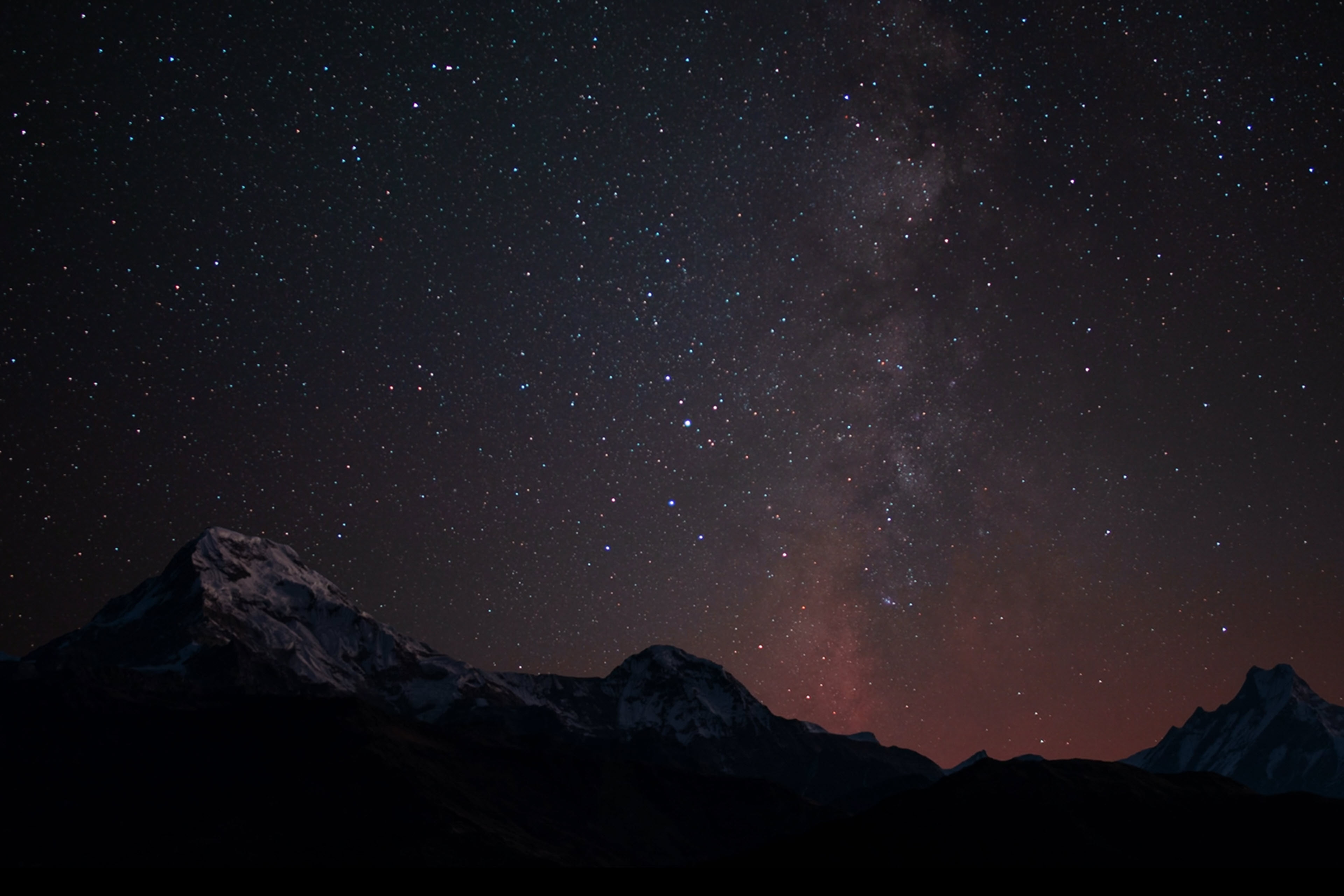This image captures a mesmerizing night sky dotted with countless tiny white stars stretching across the vast black expanse. Near the center at the bottom, a soft gradient of light pink and a hint of red and brown add a touch of ethereal beauty, suggesting the subtle glow of an unseen phenomenon. Below this enchanting sky, the landscape features a grand snow-capped mountain range with three prominent peaks—two on the left and one on the far right. These peaks stand tall against the darker background, their white snow glistening subtly. In the foreground, a shadowy silhouette of smaller hills or a secondary mountain range adds depth and mystery, cloaked in darkness and revealing no further details. The overall composition evokes a sense of otherworldly tranquility, as if capturing a moment from a science fiction scene set under an infinite, star-studded cosmos.